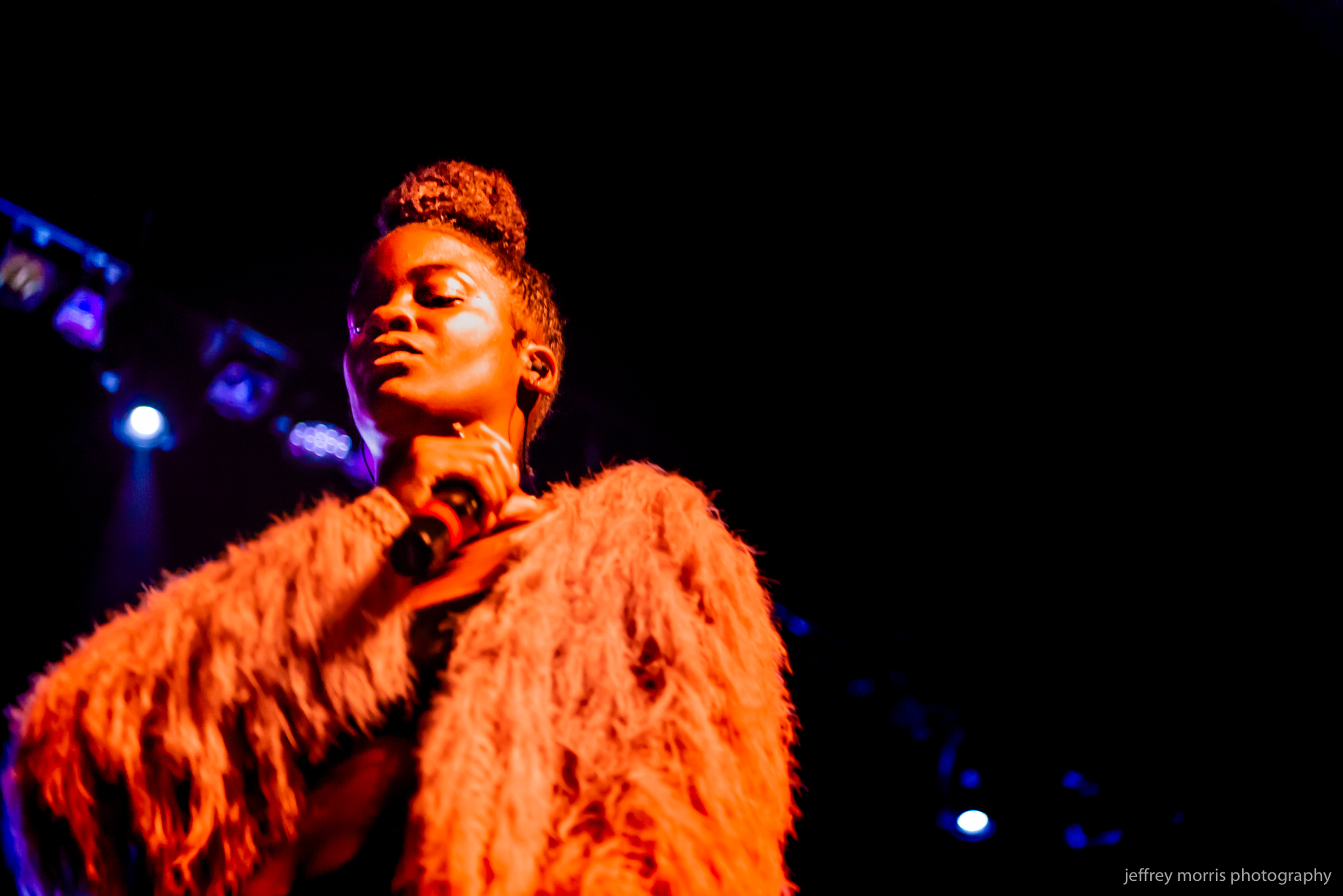The photograph captures a detailed scene of a performer, possibly a singer or pop star, holding a microphone in her right hand. The microphone, adorned with a distinctive red band at its base, is poised near her neck. The woman sports a striking outfit composed of a faux fur coat with multiple strands of fur emanating from it, paired with a black top. Her hair is elegantly styled into a black bun atop her head.

The background on the right half of the photograph is entirely black, but intricacies like scaffolding running diagonally from the top left to the bottom right corner are subtly visible. This scaffolding supports multiple spotlights aimed downwards, although the top right corner remains pitch black due to lighting and camera focus. Notably, “Geoffrey Morris Photography” is inscribed in grey transparent text in the bottom right corner of the image.

The setting appears to be a stage, possibly indoors, with a dramatic play of lights illuminating the performer against the dark backdrop, highlighting the orange-red hue of her coat, which could be due to the vivid stage lighting. The performer is additionally adorned with earplugs and a ring, adding another layer of detail to her appearance.